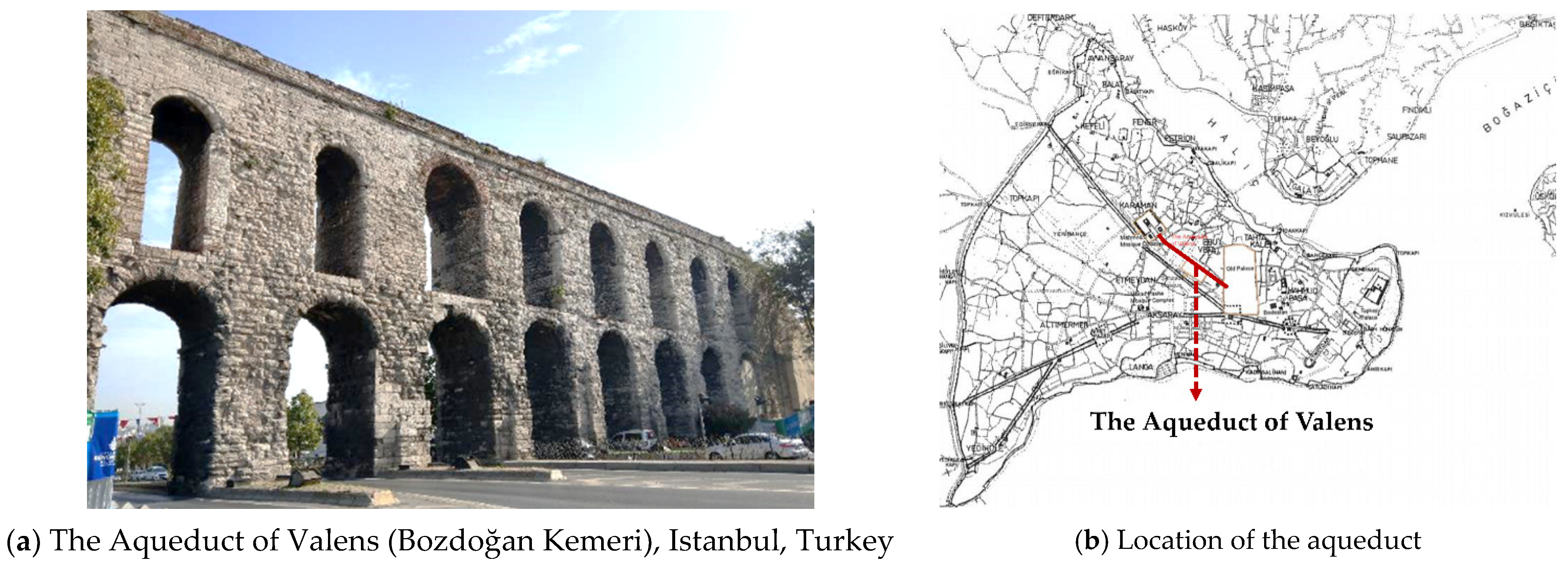The composite image features two distinct sections, labeled A and B. On the left (labeled A), there is a photograph of the Aqueduct of Valens, also known as Bozdogan Khmeri, located in Istanbul, Turkey. The aqueduct is depicted as a large, concrete structure with a series of stone arches. The arches allow for vehicular passage, visible by the cars driving through them on an asphalt road that runs beneath the structure. Above the aqueduct, the sky is a clear blue. Underneath this photograph, there is a caption that reads "A) The Aqueduct of Valens, Bozdogan Khmeri, Istanbul, Turkey."

On the right side (labeled B), there is a black and white map indicating the location of the aqueduct in Istanbul. The map includes a red line and an arrow pointing to the designated site, accompanied by text that reads "B) Location of the Aqueduct." Both images complement each other to provide a visual and geographical context of the historic aqueduct in Istanbul.